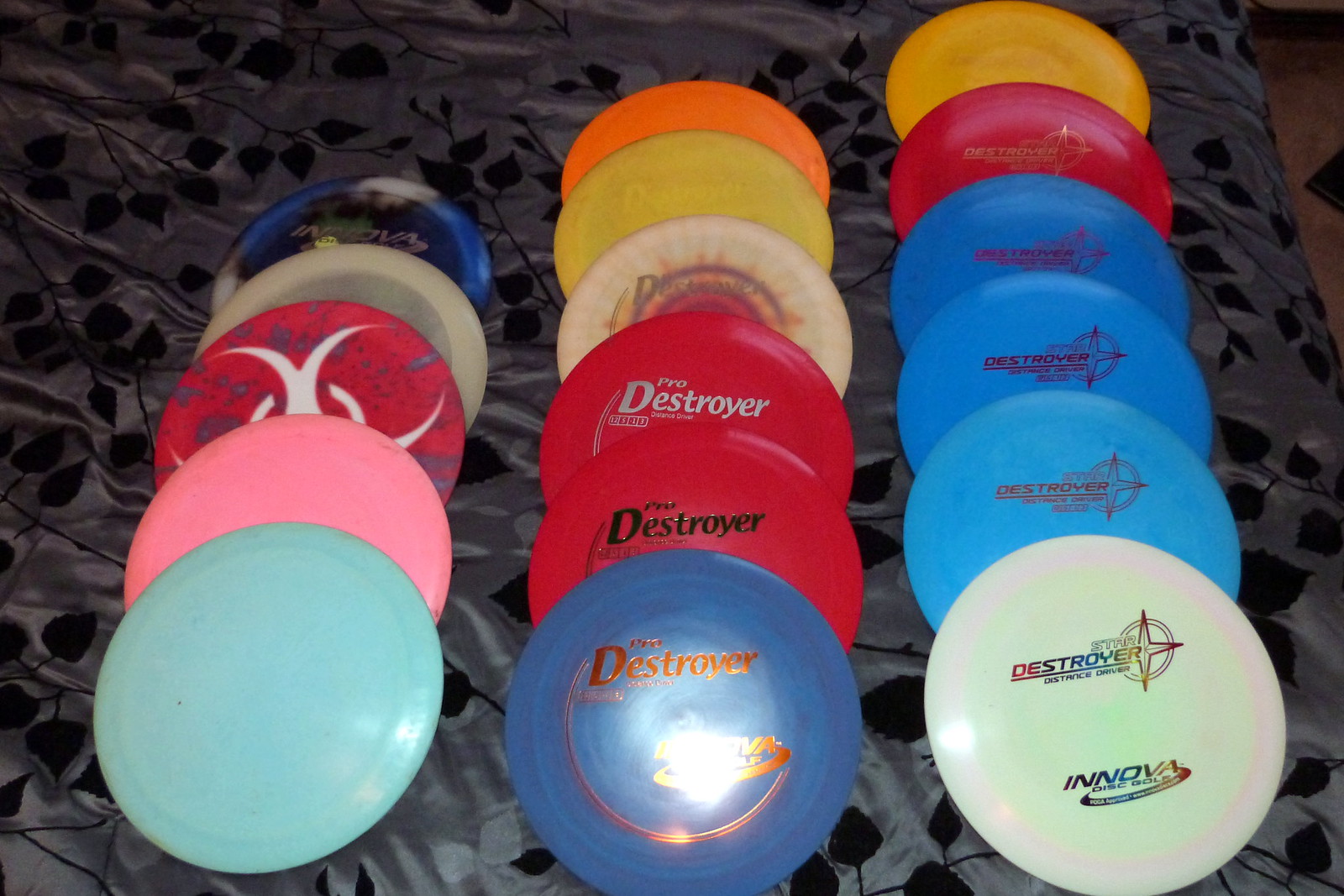This detailed image depicts a neatly arranged assortment of seventeen frisbees organized in three vertical rows on a dark gray bedspread adorned with black floral or vine patterns. The layout on the left side features five frisbees: a blue frisbee at the top, followed by a pink one, a red one with a white swirling biohazard symbol, a glow-in-the-dark disc, and a blue, black, and white tie-dyed frisbee at the bottom. The middle row showcases six frisbees: a blue frisbee at the top with "DESTROYER" emblazoned on it, succeeded by a red frisbee with the same label in black letters, another red frisbee with "DESTROYER" in white letters, a white frisbee with an orange sun design, a solid yellow frisbee, and a solid orange frisbee at the bottom. The rightmost row contains six frisbees: a white frisbee with a green center that reads "DESTROYER" in rainbow letters, followed by three blue frisbees with a star symbol next to "DESTROYER," a red frisbee with "DESTROYER," and a yellow frisbee at the bottom. The overall presentation of vibrant frisbee colors and the distinctive labeling of "DESTROYER" on several discs are highlighted against the dark, leafy-patterned bedding.